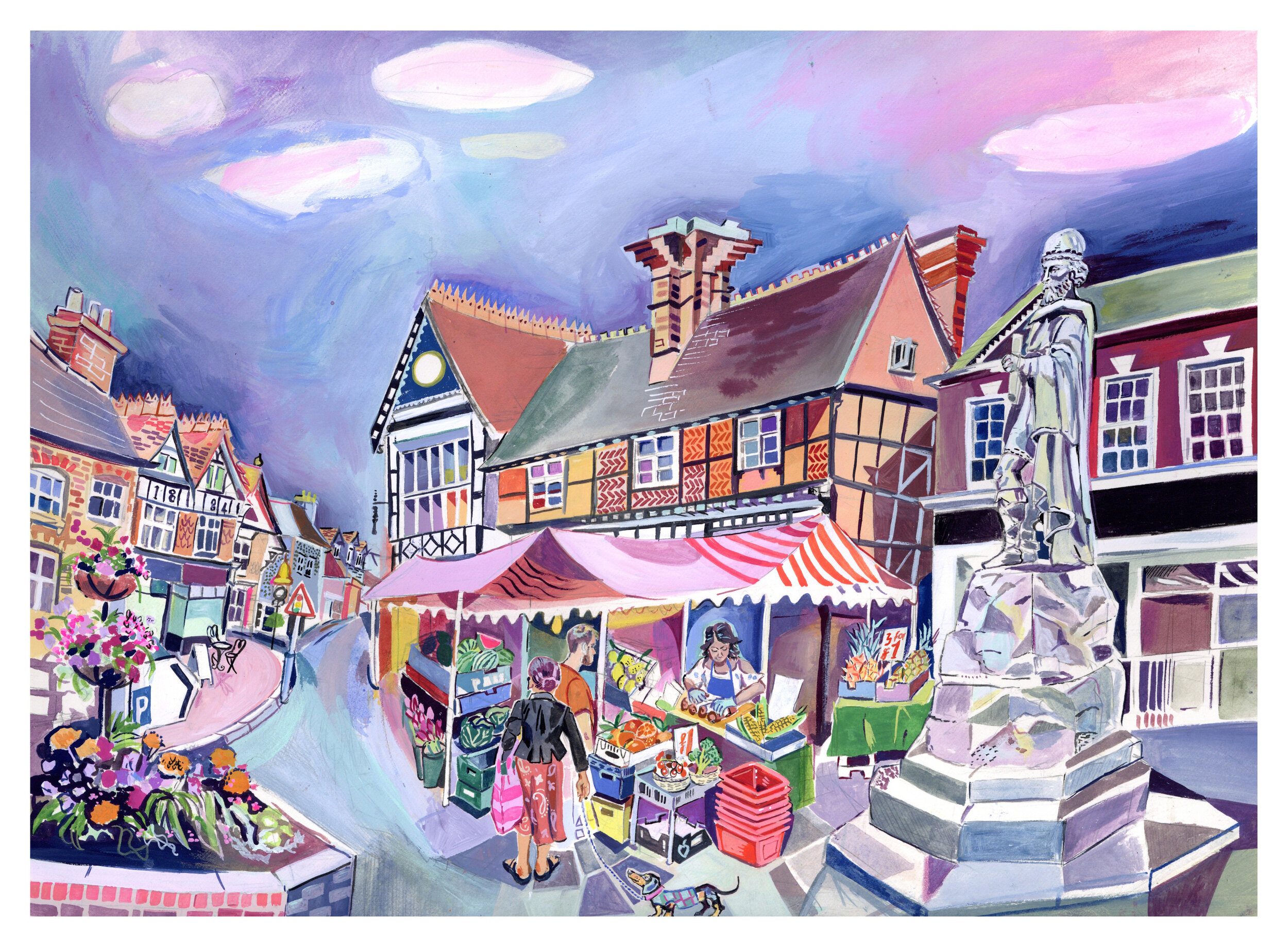This image is a realistic painting of an outdoor market in a charming European village. The scene is set in a colorful market street surrounded by quaint, gingerbread-style houses, each painted in vibrant hues. The sky above is a captivating blend of purplish-blue and pink, intermingled with white and pink clouds, creating a dreamy backdrop.

In the bustling center of the market, a dark-skinned woman wearing a blue apron stands behind a stall selling various foods. Her stall is filled with an assortment of vegetables and there are red shopping baskets available for patrons. Engaging with her are two customers: a man in an orange shirt and a woman dressed in a black top and red blouse, carrying a pink bag. Accompanying them is a charming dark-colored wiener dog adorned with spots and a red collar.

On the right-hand side of the scene, a prominent statue of a man on a large pedestal adds a sense of history to the market square. To the bottom left, there's a beautiful arrangement of orange, red, and pink flowers, blooming in staggered baskets.

This detailed depiction captures the essence of a lively farmer's market, highlighting the interaction between vendors and patrons, with a picturesque and almost medieval architectural setting.